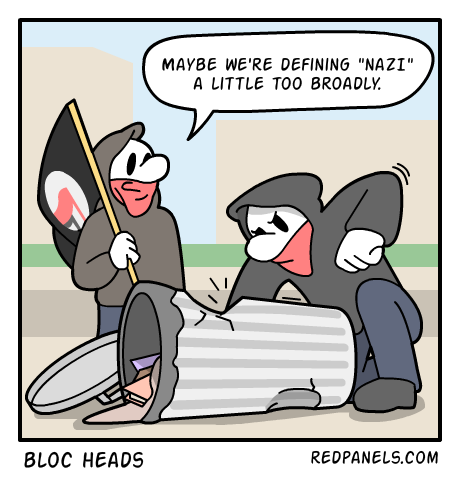The image depicts a frame from a comic strip featuring two cartoon-style men with fair skin and black eyes, each wearing a gray hoodie, blue pants, and gray shoes. Both have red bandanas covering their mouths. They are positioned next to a tipped-over garbage can, spilling its contents. One of the men is holding a black flag with a white circle and a red object in the center. A speech bubble above him reads, "Maybe we're defining Nazi a little too broadly." The style is distinctly comic-like, with the characters centered. The bottom left corner of the frame includes the text "Blockheads," while the bottom right corner notes the web address "redpanels.com." The color palette includes light blue, black, white, gray, yellow, red, and purple.